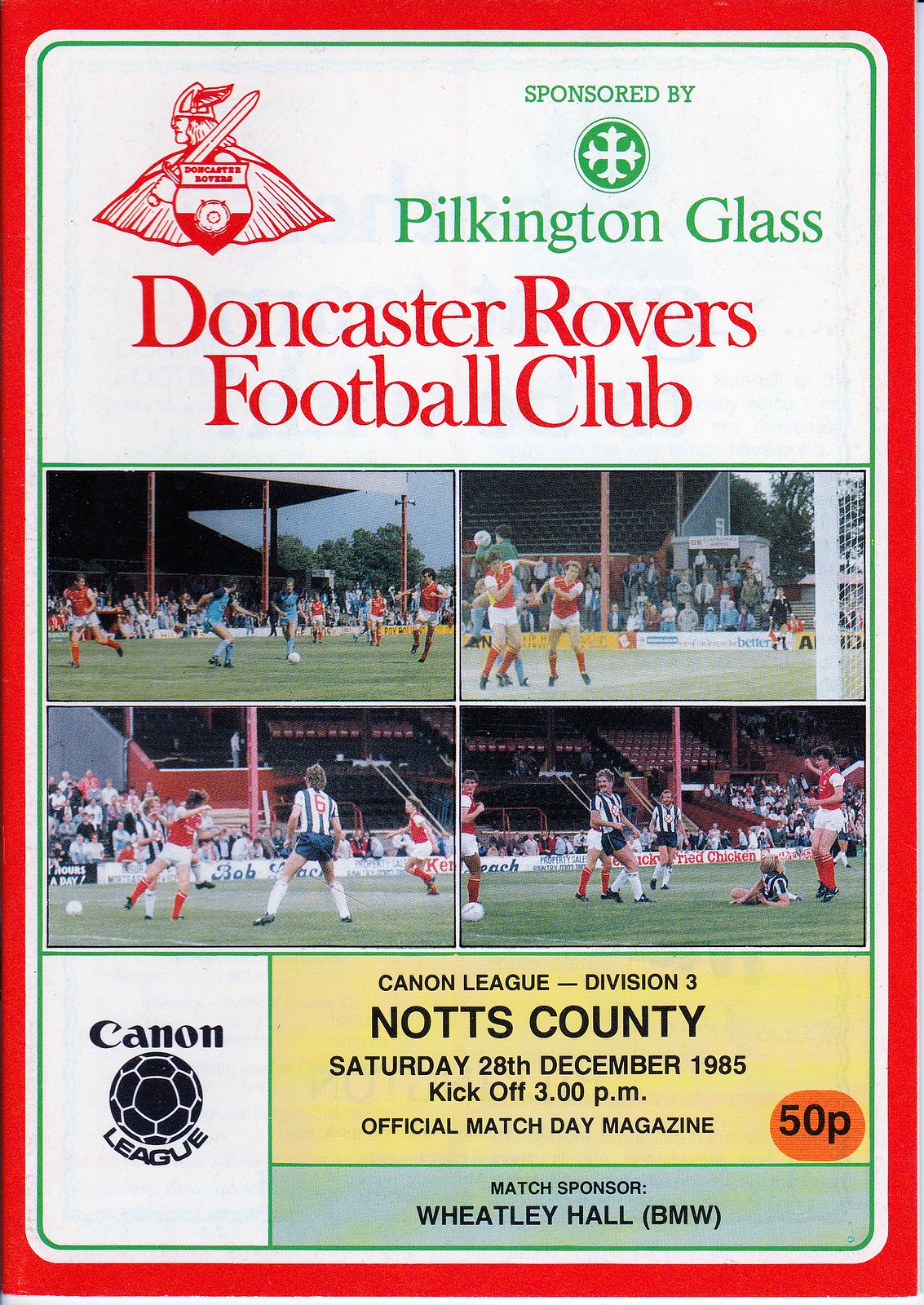This image is a detailed front cover of a promotional program for a Doncaster Rovers Football Club match held on Saturday, December 28, 1985. The program announces a Division III Cannon League match against Knotts County, with kickoff scheduled for 3 p.m. The cover design features a prominent red border and a top white text box displaying the team's logo—a Viking holding a sword in front of a shield—along with a text indicating sponsorship by Pilkington Glass, written in green next to a Celtic cross-like logo. There are four central photographs of players in action, all featuring teams in red jerseys, with some opponents in blue or striped jerseys. Below these images, additional information is provided: the Cannon League logo with a black soccer ball, the match sponsor Wheatley Hall BMW, and the price of 50 pence for the program. The overall design incorporates color blocking in yellow and green, reinforcing the sponsorship details and event information.